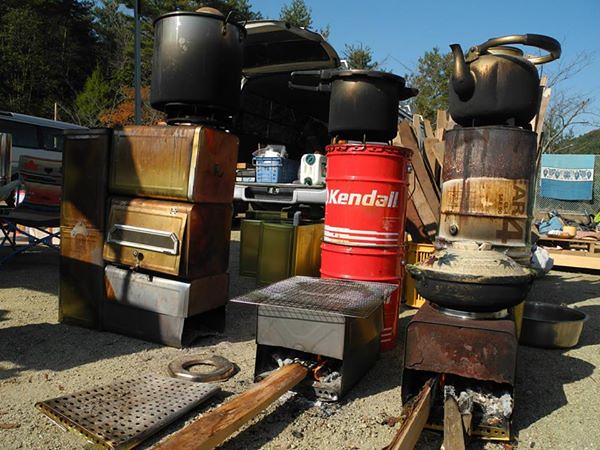The photograph, taken outdoors on a bright, sunny day under a vivid blue sky with distant green trees, showcases a peculiar assortment of metal objects displayed on a sidewalk. Prominently, several industrial pieces, which resemble eclectic handmade stoves and wood-fired ovens, capture attention. These stoves, some old and rusted with flames flickering from their coal beds, are designed for wood at the base. One stove stands out with its modern, stainless steel or aluminum construction, topped by a flat grate. Surrounding these stoves are numerous metal barrels, including a striking dark orange and white one labeled "Kendall." Resting on top of the barrels and scattered across the area are large, black cast iron pots and kettles, including a notable teapot with a spout. Additional items like metal boxes and various used metal components add to the cluttered, makeshift environment, creating an impression of a rustic scrapyard. Further in the background, a blue banner or towel hangs messily, contributing to the overall disordered yet intriguing scene.